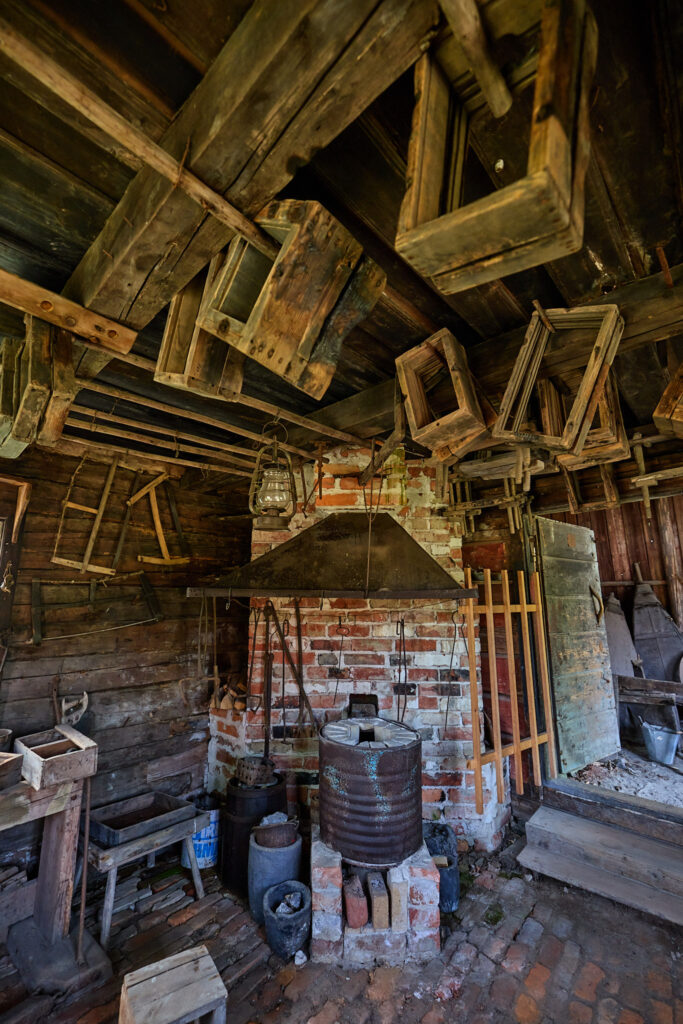The image depicts a rustic, seemingly dilapidated room, primarily constructed of red brick and wood. The brick walls and flooring are visible, with a brick fireplace or oven as the focal point in the background. Various wooden elements are scattered throughout the space, including rafters from which canvases hang, multiple planks, small stools, and a broken door. The ceiling also features wooden beams. Within the room, there is a combination of both metal and wooden objects, such as metal barrels and drums, a large metal vent as part of a stove setup, and several wooden boxes and cabinets. A large metal barrel sits atop the stove, reinforcing the room's rough, primitive atmosphere. Stairs and an open door on the right side of the image suggest a connection to the exterior, enhancing the sense of an old, worn-out structure.